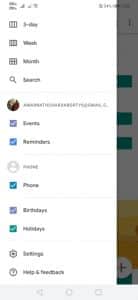This image is a blurry screenshot of a menu page within a mobile application. The lower portion of the screen features a horizontal gray navigation bar with three outlined icons. The first icon resembles a network connection symbol with a large circle on the left connected to two smaller circles on the right. The second icon looks like a circular button, while the third one appears to be either a square or rectangular button.

The main section of the menu mimics the layout found in social media apps, such as Facebook. It begins with several calendar view options, each represented by an icon followed by text. The first three options include calendar icons with corresponding text labels: "Three day," "Weekly," and "Monthly." Below these options, there's an icon of a magnifying glass with the text "Search" next to it. A thin gray dividing line separates this section from the next.

Further down, there is a circular avatar icon, which is partly tan and partly maroon, indicating a user profile. The profile name is long and blurry, trailing off with an ellipsis as it gets cut off towards the right. Underneath the profile section, a purple square with white text reads "Events," followed by a similar blue square also with white text, labeled "Reminders." 

Another dividing line follows, beneath which lies a generic profile avatar icon—a gray circle with a white portrait in the center. The accompanying text is not legible. Directly below, there’s a teal blue box with a white check mark and the text "Phone." Another dividing line separates this from a light purple-gray box, also with a white check mark, labeled "Birthdays." Following this is a green box with a white check mark and the text "Holidays."

At the bottom of the menu, there’s a settings icon accompanied by the text "Settings," and a question mark inside a circle with the text "Help and feedback."

The dropdown menu occupies about 90% of the screenshot’s width. The remaining 10% displays a grayed-out or blacked-out background of another app, possibly with a white background initially. In this area, three rectangular boxes are faintly visible to the right of the “Search,” “Events,” and “Reminders” rows. The bottom right corner also reveals part of a Google Plus icon, specifically the right two-thirds of the circle.

Overall, the image captures a densely-packed navigational menu with multiple sections delineated by icons, text, and dividing lines, offering various functionalities related to calendar views, user profiles, and app settings.